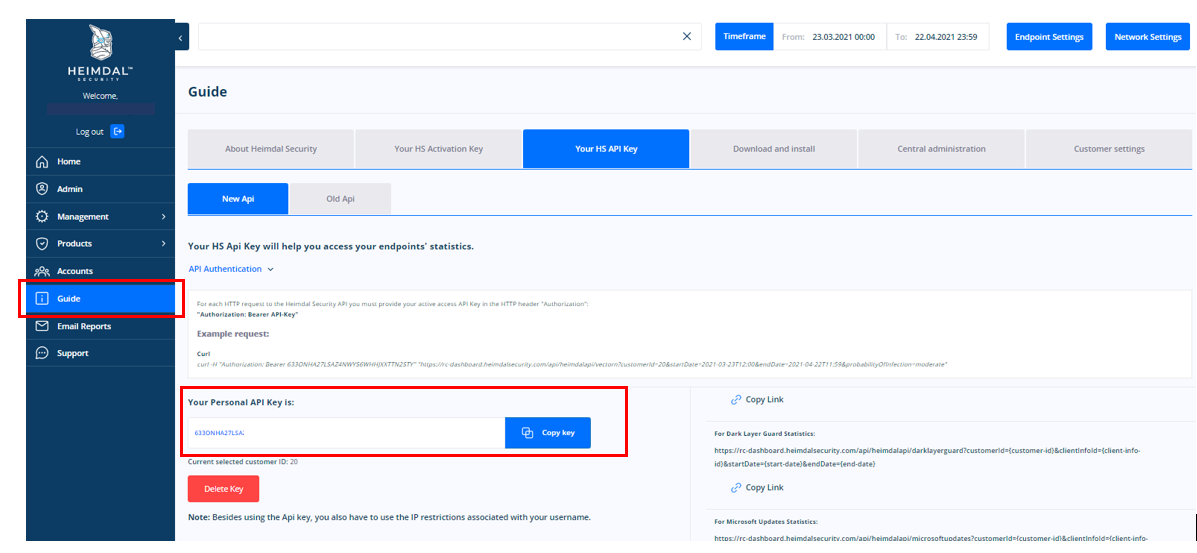The image depicts a detailed screenshot of the Heimdall website interface. In the upper-left corner, the Heimdall logo is prominently displayed, followed by a logout button. Directly below, a vertical column features several menu tabs. The sequence of the tabs includes Home, Admin, Advisors, Management, Products, Accounts, Guide, Email, Reports, and Support. The text of these tabs is very small and somewhat difficult to read.

At the top center of the interface, there's a search bar positioned beside additional menu options such as Time, Timeframe, and two text boxes for specifying a date range or other parameters. Further menu items include Endpoint Settings and Network Settings.

Beneath these, the main content of the interface is organized, beginning with a header labeled "Guide". This section contains six menu options. The currently selected option is "HSAPI key". Other menu items include New Age, Old Age, and a box highlighted at the bottom that displays "Your Personal API Key Is". The overall layout is clean and structured, designed for easy navigation despite the small text.